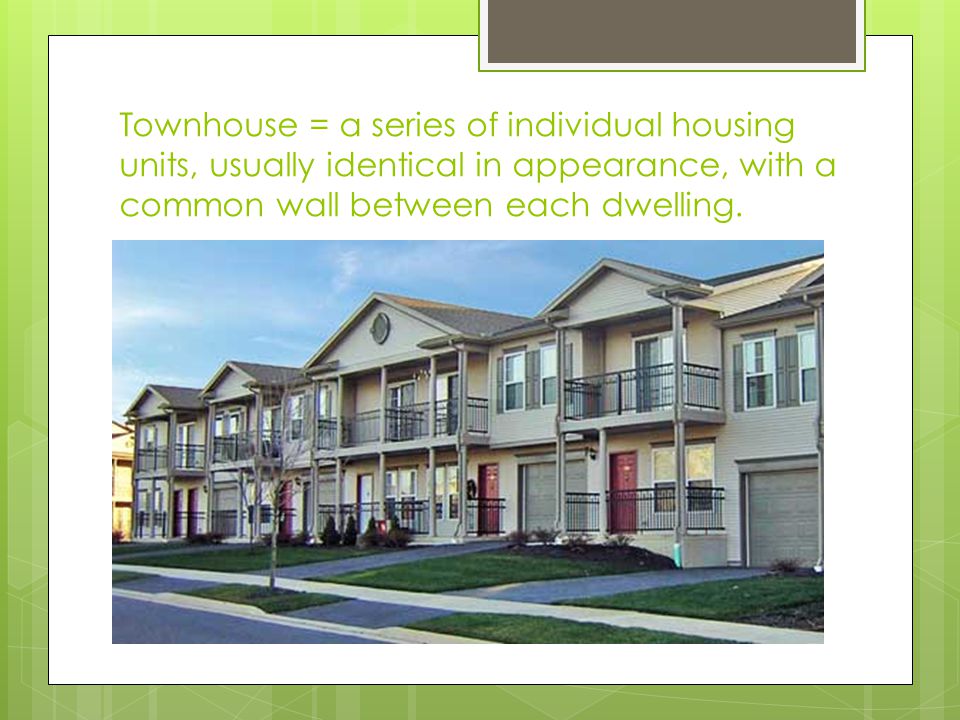The image is a presentation slide primarily designed to define a townhouse. It features a green-outlined border framing a white background. At the top of the slide, in bright green Century font text, the description reads: "Townhouse equals a series of individual housing units, usually identical in appearance, with a common wall between each dwelling." The main photograph, positioned towards the bottom center, showcases a row of four or five connected townhouses, depending on where the image is cut off. Each townhouse has two levels, a balcony with black railings, beige rooftops, cream-colored exteriors, and red front doors. Visible in the foreground are driveways, some grass patches, and a street at the bottom left. Additionally, there is a gray cut-off box in the top right corner of the slide, and the overall style suggests it is part of a PowerPoint presentation. The color scheme includes green, black, white, gray, red, and blue.